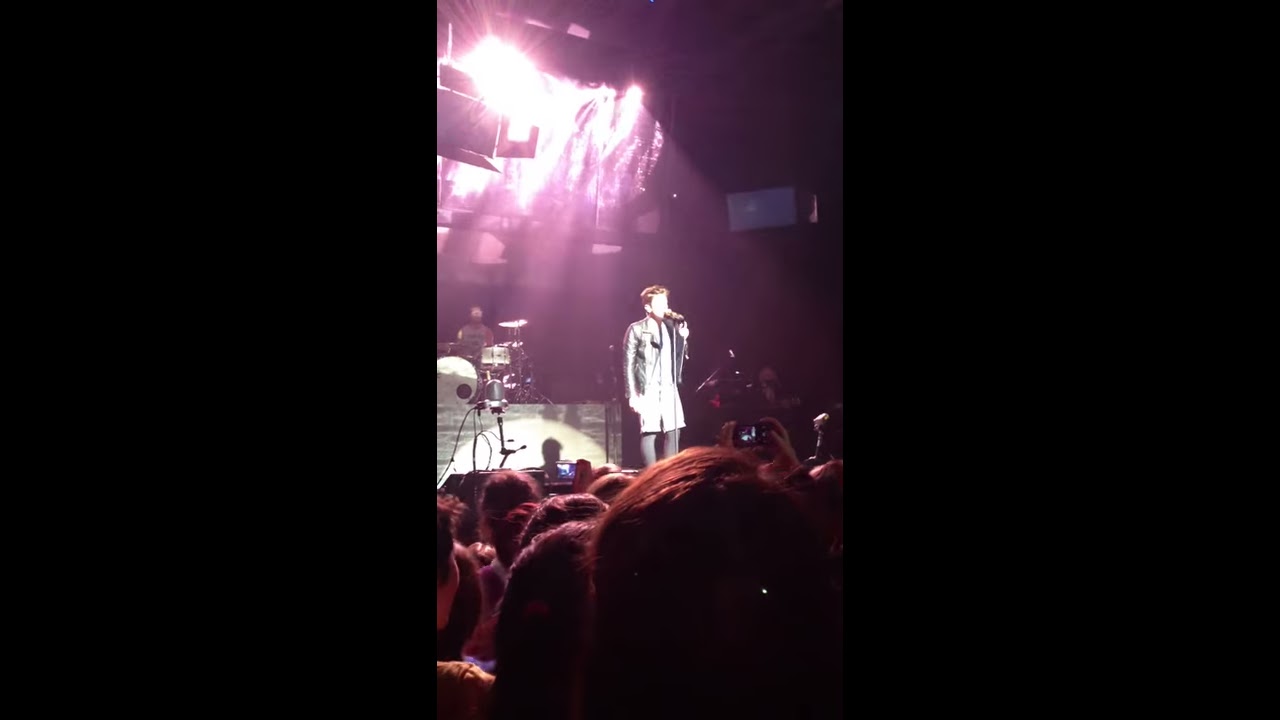This image, slightly blurry and vertical like a cell phone snapshot, captures a singer on stage at a concert. The performer, positioned directly in the center, is wearing a leather jacket and possibly leggings, with short hair, making it difficult to discern specific features or if they are a known artist due to the lighting. Bright stage lights shine from behind, obscuring more detail. Behind the singer, a drummer is visible with his back turned, among a set of drums. The photo is taken from within the crowd, where silhouetted heads and raised cell phones are recording the event. The scene is framed with dark borders, and a mix of colors like brown, tan, white, black, gray, purple, and pink add depth to the venue, suggesting either an indoor or outdoor setting. Overall, while specifics are blurred, the image unmistakably conveys the dynamic atmosphere of a live concert.